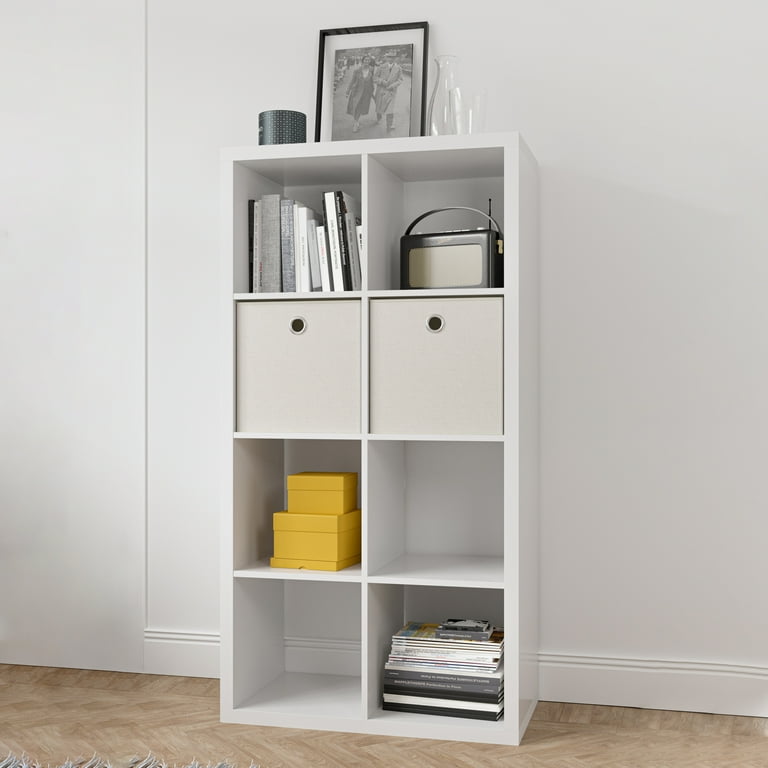This photograph, taken indoors, captures a white wooden bookcase against a white wall and set on a light to dark brown wood grain floor. The bookcase consists of eight square cubbies arranged in four rows of two. Sitting atop the bookcase is a black-framed, black-and-white photo of a man and a woman, flanked by a clear glass vase and a cylindrical object that appears to be a small speaker.

The top row of cubbies features a small portable TV on the right and a series of books on the left, though the titles are unreadable due to the focus. The second row contains two closed canvas boxes with grommets, serving as handles. The third row shows a set of small yellow boxes on the left, with the right cubby remaining empty. The bottom row features an empty cubby on the left and an assortment of magazines on the right.